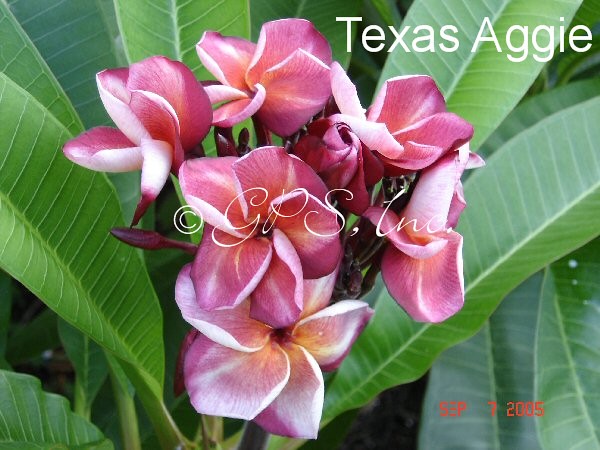This image features a vivid outdoor scene showcasing a plant with large, oval-shaped green leaves prominently displaying visible veins. Interspersed among these leaves are six fan-shaped flowers, mostly pink with hints of white and a touch of orange in the center. Some buds are visible, indicating flowers that are still forming. In the upper right corner, the text "Texas Aggie" in slender white cursive identifies the plant. Superimposed in the center of the photograph, the copyright notice "GPS Inc." is clearly marked. The date "September 7, 2005" is displayed in the lower right corner in yellow text. The overall composition is bathed in natural light, enhancing the vivid green of the leaves and the delicate hues of the flowers.